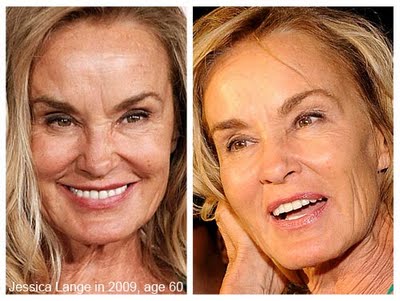The image consists of two side-by-side photographs of actress Jessica Lange, taken in 2009 at the age of 60. The left photograph, labeled "Jessica Lange in 2009, age 60," shows her looking directly at the camera with a warm, white-toothed smile. She has dark eyebrows, hazel-green eyes, and flowing blonde hair cascading down from her face, visible from the neck up. In this image, her Caucasian complexion is complemented by her pleasantly expressive eyes and smile. The right photograph features Jessica Lange in a slightly different pose; she is tilting her head and resting it gently on her hand. Despite the subtle variation in the angle and slightly shorter appearance of her hair, her distinct blonde locks, dark eyebrows, green eyes, and pink lips remain consistent. Visible from the neck up with some wrinkles noticeable around her neck, she maintains a slightly smiling, happy, and engaged expression. Both images are close-ups with a dark background, highlighting her captivating presence and consistent peaceful demeanor.